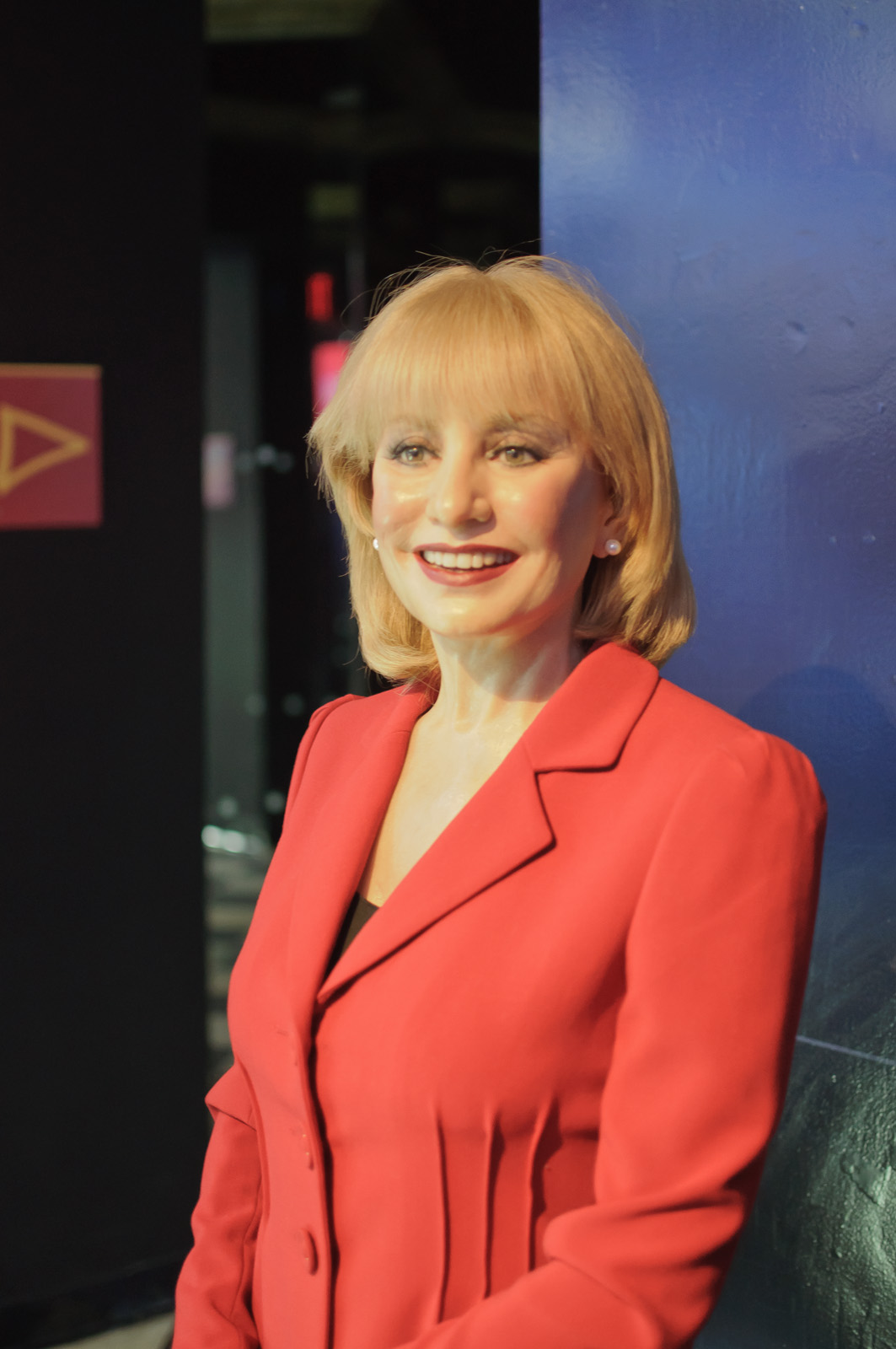In the image, a woman is centered, standing inside a building, illuminated by a spotlight against a backdrop of contrasting colors. The wall behind her is primarily navy blue transitioning into gray towards the bottom. To her left, there is a dark wall marked by a red sign with an orange arrow, suggesting an event setting, possibly a stage or backstage area. The woman, who resembles a younger Barbara Walters, has shoulder-length, light blonde hair with bangs framing her face. She is smiling, looking slightly to the side of the camera, wearing red lipstick. Her attire consists of a coral-colored blazer with three pleats down the front and two buttoned-up buttons, under which she dons a black tank top or similar shirt. She accessorizes with small pearl earrings.